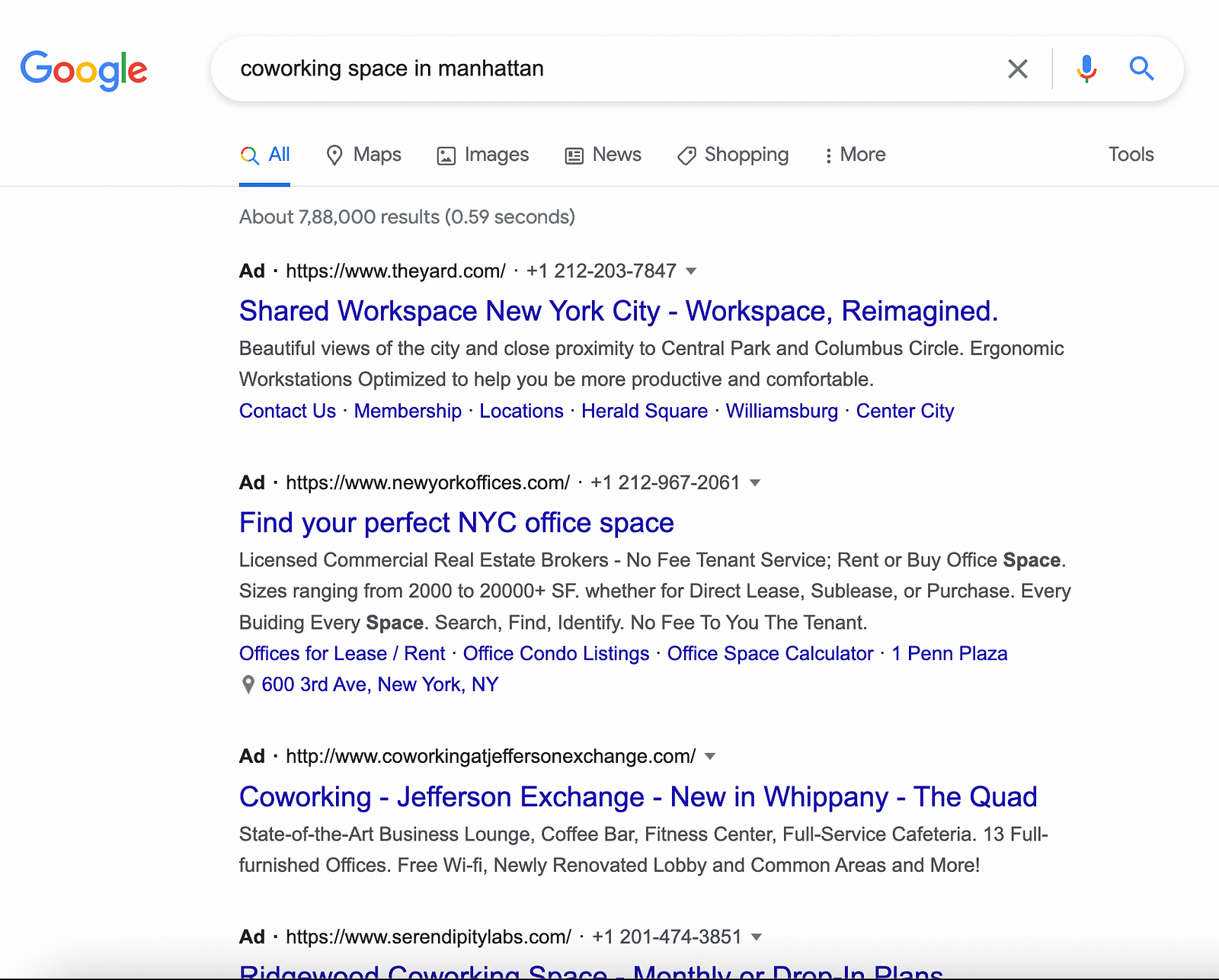The image features a Google search page interface. In the upper left corner is the iconic Google logo composed of vibrant letters: a large blue "G", a red "O", a yellow "O", a blue "G", a green "L", and a red "E". Adjacent to the logo, there's a search bar with the text "co-working space in Manhattan" entered in it. On the right-hand side of the search bar are the icons for closing the search (an 'X'), voice search (a microphone), and initiating the search (a magnifying glass).

Beneath the search bar, a navigation row offers various categories: "All," "Maps," "Images," "News," "Shopping," "More," and "Tools." Below this, on the left side, is an advertisement marked "Ad," accompanied by a URL. The advertisement features a headline in blue text reading "Shared Workspace New York City Workspace, Reimagined." It highlights facilities with beautiful city views, proximity to Central Park and Columbus Circle, and ergonomic workstations designed for productivity and comfort. The ad also mentions sections such as "Contact Us," "Membership," "Locations," "Herald Square," "Williamsburg," and "Center City."

Another listing marked as an "Ad" with a URL follows, promoting "Find your perfect NYC office space" in blue text. It describes options and services provided by real estate brokers. Farther down, another sponsored listing with a URL mentions "Co-working Jefferson Exchange new in WHIPPANY – the Quad," followed by additional details.